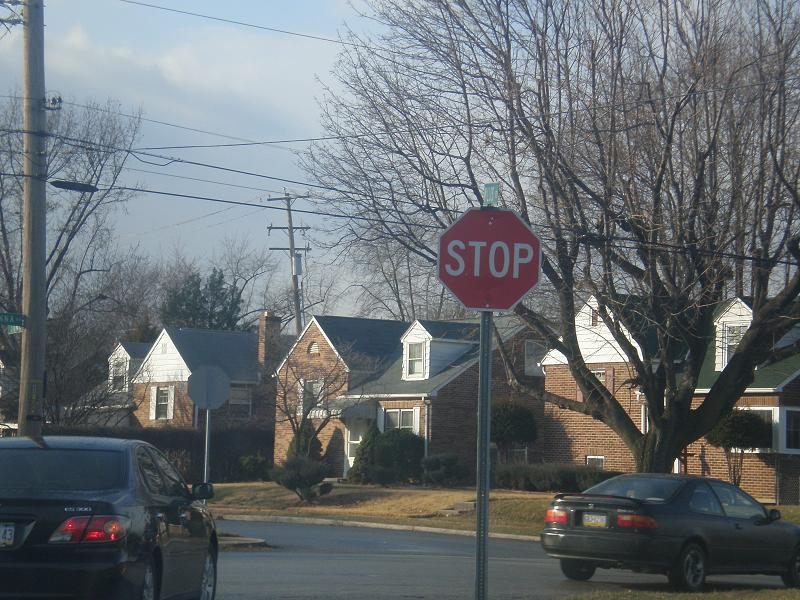The image captures a late afternoon scene in a neighborhood dominated by a stop sign mounted on a gray metal pole, displaying the word "STOP" in white letters against its red backdrop. At the bottom left, a black car can be seen with its brake lights illuminated. Another black car is parked along the curb to the right. The background features three nearly identical, two-story brick houses with white-trimmed windows and doors. These houses each have dormer windows jutting out from their dark green-black roofs. The front yards display a mix of green shrubs and patches of dead, brown grass. Large trees with bare branches, indicating they are out of leaf, stand tall amidst the houses along with wooden telephone poles carrying black power lines. Above, the sky is a mix of blue and gray clouds, adding to the serene yet somewhat desolate atmosphere of the neighborhood.